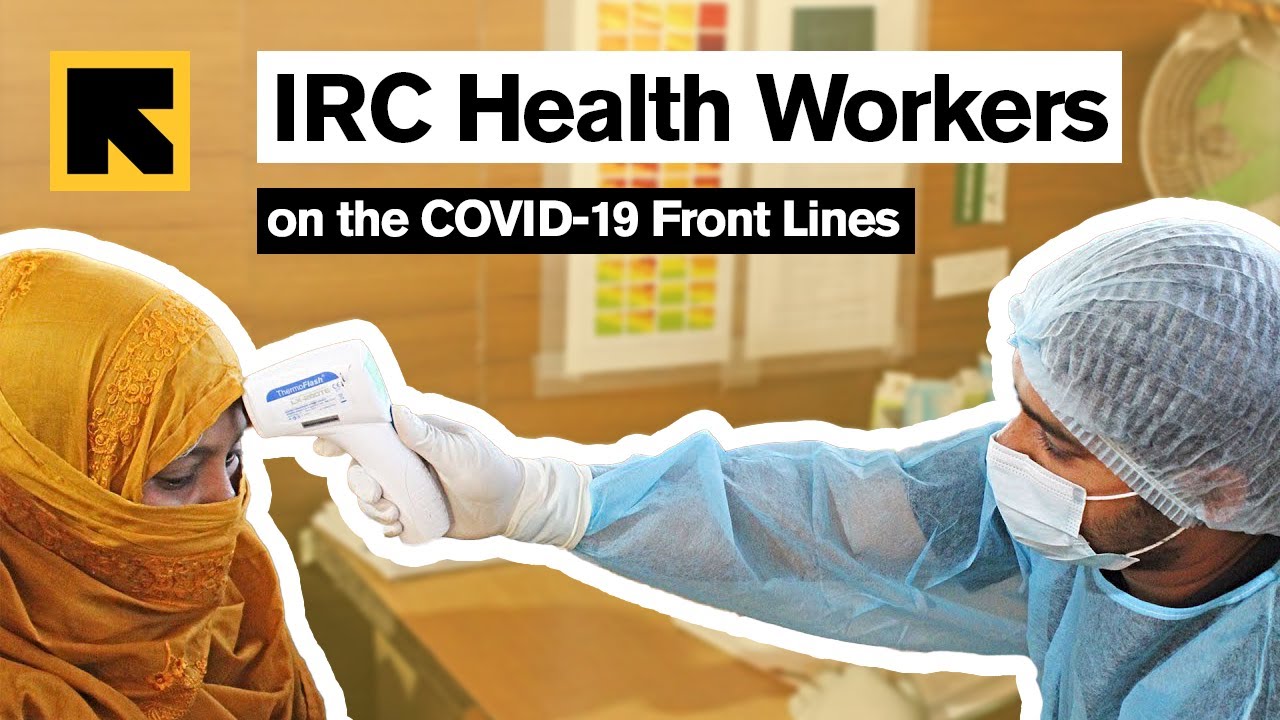This rectangular image appears to be a screenshot and prominently features a scene set in a healthcare environment. On the right side, a medical worker, clad in a blue transparent protective suit, latex gloves, a surgical mask, and a hairnet, is depicted. He is reaching over to the forehead of a woman with a handheld thermometer gun, a device used to measure body temperature. The woman is wearing a gold-colored hijab, which covers her head. Both their bodies are digitally outlined in thick white, creating a striking visual effect. At the top of the image, there is a rectangular text box with the words "IRC Health Workers" in black text. Below this, a smaller black box with white text reads "On the COVID-19 Front Lines."